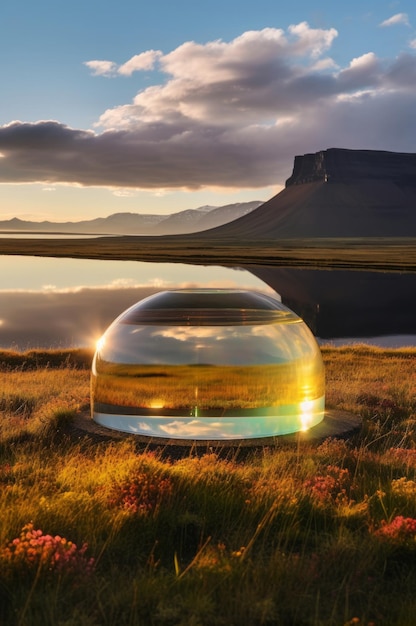In this vibrant daytime outdoor photograph, a pristine, dome-shaped glass or crystal structure takes center stage, positioned on a dark, flat pedestal. The object, reminiscent of an upside-down glass bowl filled with water, reflects and refracts the surrounding landscape with remarkable clarity. The sunlight, streaming in from the left, casts a shimmering reflection to the bottom right of the dome. It stands in a grassy field, dotted with delicate light pink wildflowers, suggesting a late-year, greenish-brown hue to the grass.

Directly behind this scene, a vast, mirror-like lake stretches out, its pure, unblemished surface adding a serene element to the composition. Beyond the lake, a dramatic mesa rises sharply, its flat silhouette contrasting against dark gray clouds that gather above it. The top right of the image features glimpses of blue sky peeking through the clouds, adding depth and a touch of brightness to the otherwise moody backdrop. The overall scene is one of natural beauty and tranquil reflection, with the crystal-clear dome acting as a focal point that draws the viewer into the expansive, picturesque landscape.